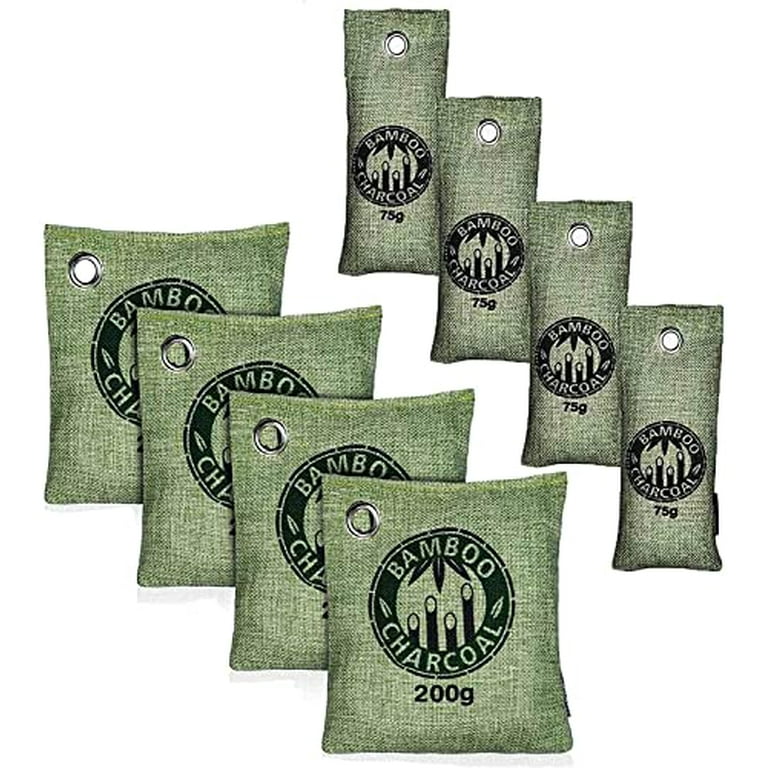The image showcases bags of bamboo charcoal in two distinct sizes and shapes. In the bottom left corner, there are four square-shaped bags, arranged in a cascading manner from front to back. These larger bags are made from a light green, sack-like material and feature a central black circle logo. The words "Bamboo Charcoal" and "200g" are printed on the front, with the bags sequenced one behind the other. In the top right corner, there are four smaller, rectangular bags, aligned side by side but staggered like steps, with each subsequent bag positioned halfway up the previous one. These 75g bags share the same light green color and black circle logo, also bearing the "Bamboo Charcoal" label. Both types of bags have metal grommets, suggesting they can be hung, and are designed with a natural, earthy aesthetic, prominently displaying their weight and bamboo charcoal content.